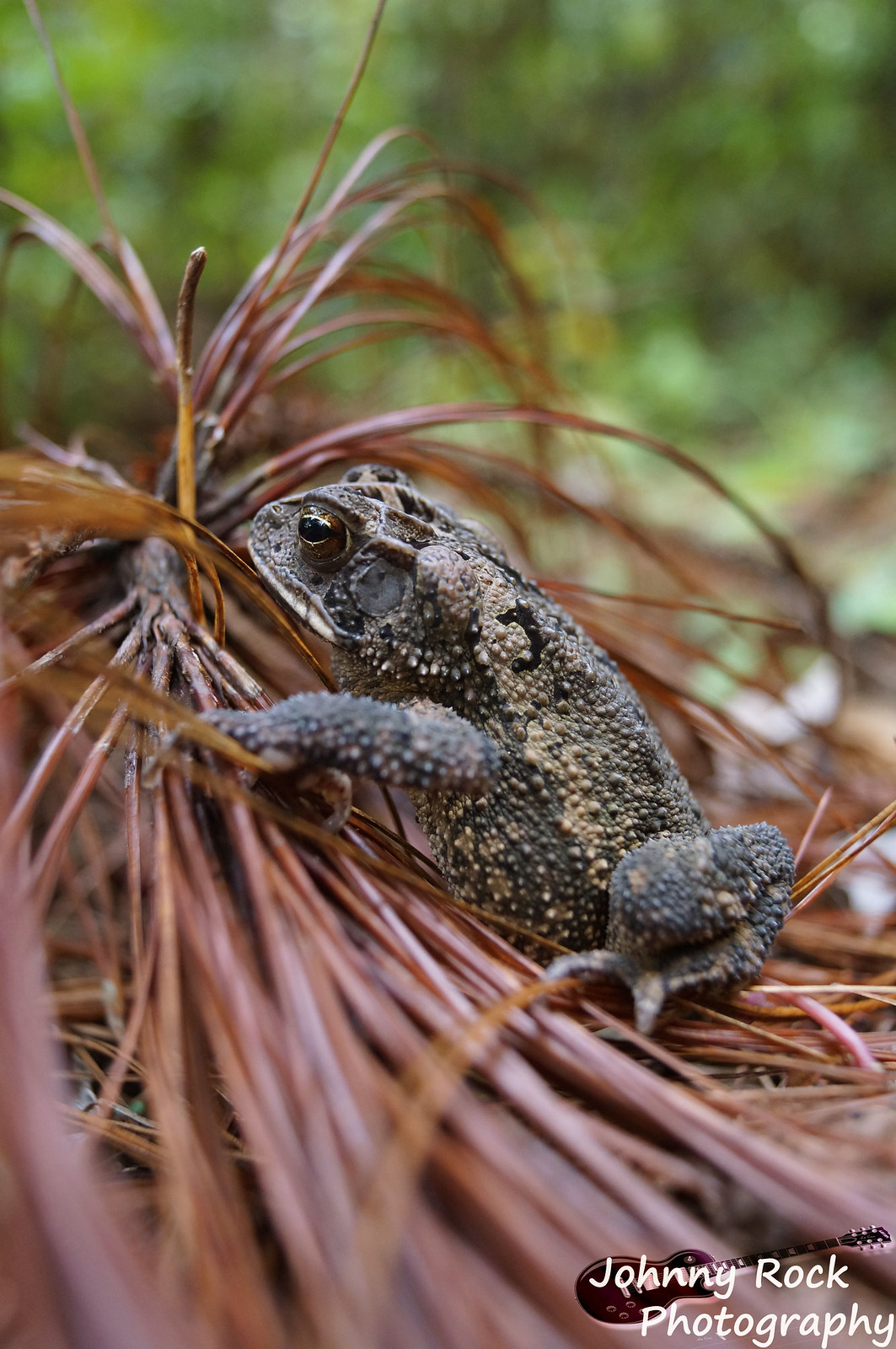The photograph features a close-up, side view of a large frog, possibly a toad, situated prominently in the center. The amphibian is predominantly black and brown with distinctive, textured spots scattered across its skin. One eye and the legs on its side are visible, emphasizing the animal's detailed, bumpy texture. The frog rests on a cluster of shiny, thin, brown reeds or grass, some of which extend upwards like fronds, suggesting a wet environment. The background is blurred with a greenish hue, hinting at foliage and creating a bokeh effect that indicates a bright, daytime setting. In the bottom right corner of the image, there is a small, brown guitar icon displaying the text "Johnny Rock Photography" in white letters superimposed over it.